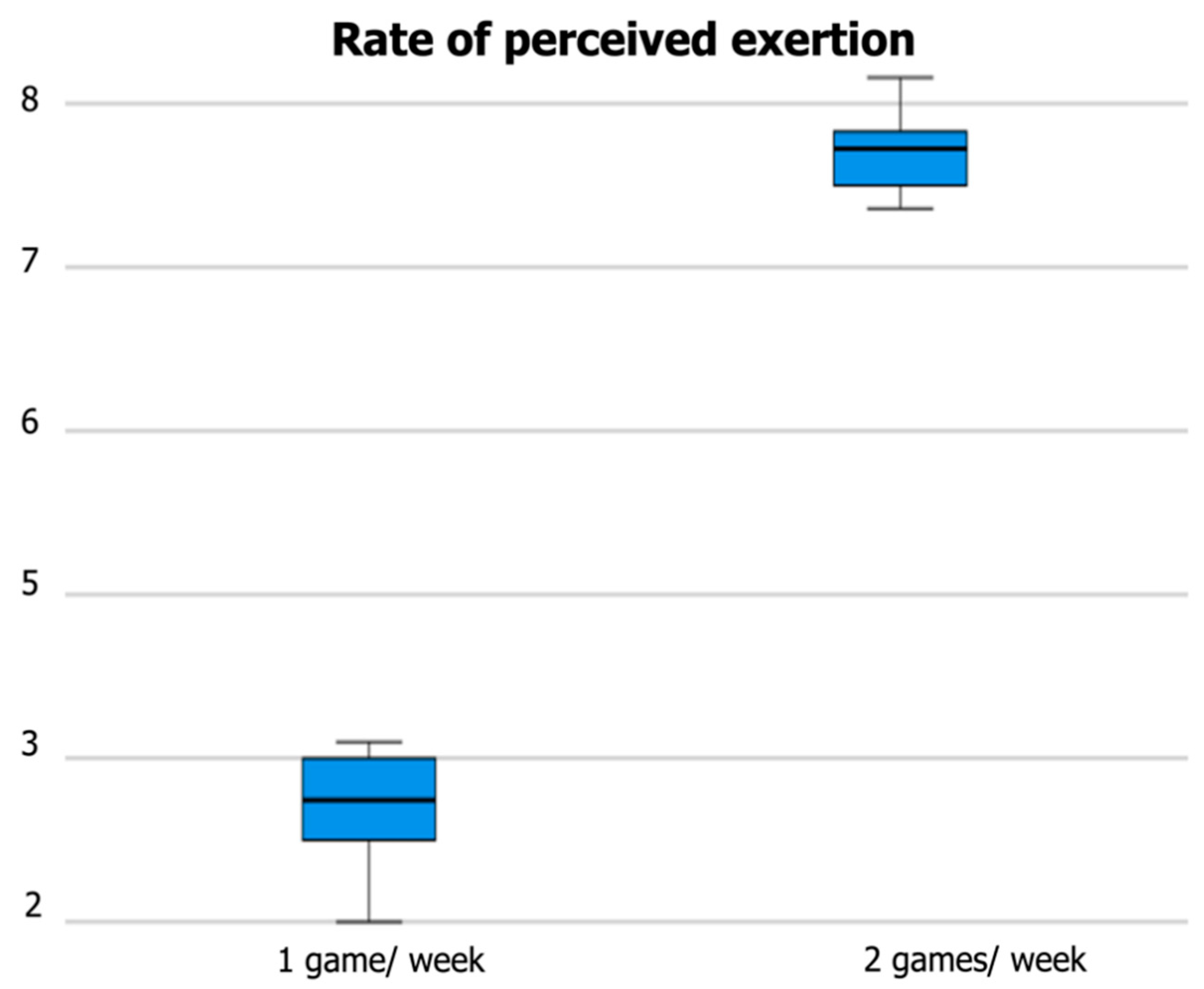The image displays a well-structured graph titled "Rate of Perceived Exertion," using Tahoma font. Along the y-axis, numbers 2, 3, 5, 6, 7, and 8 are presented vertically from bottom to top, each aligned with light gray horizontal lines traversing the graph. The x-axis compares "1 game per week" and "2 games per week." A light blue rectangular bar corresponds to "1 game per week," reaching up to 3, slightly extending beyond it with a thin horizontal black line through the middle. The bar for "2 games per week," also in light blue, stretches between 7 and 8, with a horizontal black line starting at 7 and extending just above 8. The graph effectively contrasts the exertion levels between playing one and two games per week.